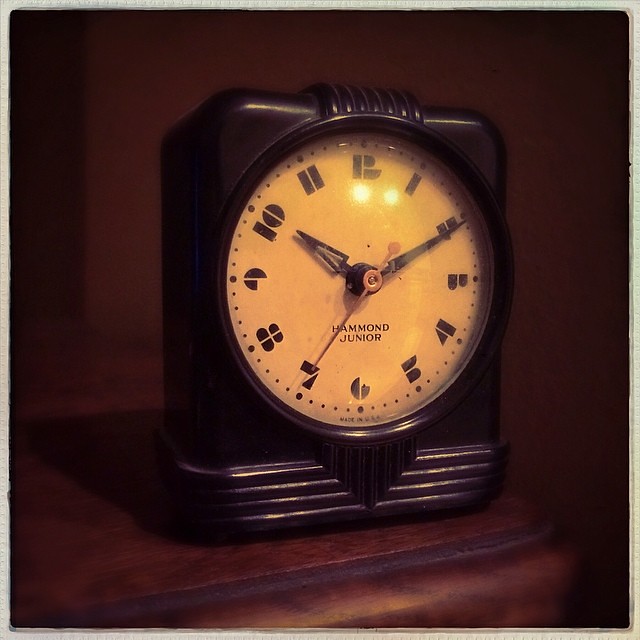This image features an angled view of a vintage, square-shaped clock with a notably thick frame. The clock's sides are impressively wide, adding to its robust appearance. Dominating the scene, the clock face is exceptionally large and features bold, block-style numerals instead of Roman numerals, offering a classic yet modern touch. The hour hand is uniquely designed like an arrow with a cut-out center, while the minute hand is sleek and sharp, reminiscent of a blade. A gold second hand adds a touch of elegance against the ivory-colored clock face. Towards the bottom center of the face, "Hammond Jr." is prominently displayed, indicating the brand or model of the clock. The clock's casing looks to be made of dark brown wood or possibly a high-quality brown plastic, exuding a rich, vintage charm. It is positioned on the right edge of a dark wooden table, adding to the antique aesthetic of the scene.